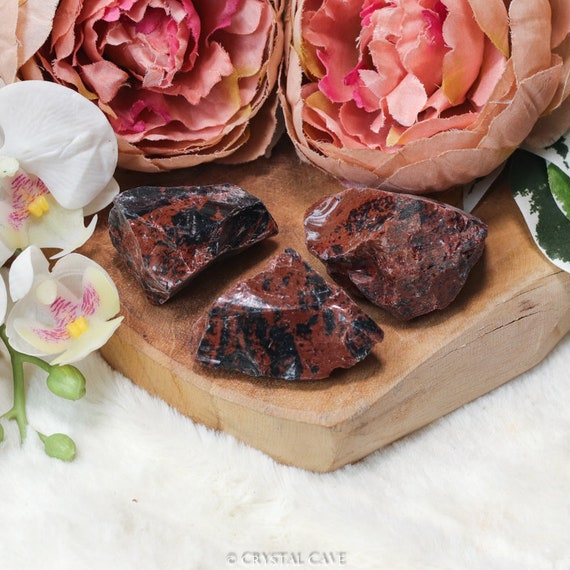The image depicts a stylish product photograph showcasing three jagged and pointy stones, potentially obsidian, with a shiny yet rough surface in shades of reddish-brown and black. These stones rest on an asymmetrical, polished slab of wood. The entire arrangement is set atop a plush, white, faux fur rug. To the left, there's a sprig of white flowers with pink and yellow centers and green stems with buds. Above the stones, two pink roses add a touch of color. The background includes speckled leaves in dark green, light green, and white hues. A watermark reading "Crystal Cave" is visible at the bottom of the image, indicating the brand or photographer.